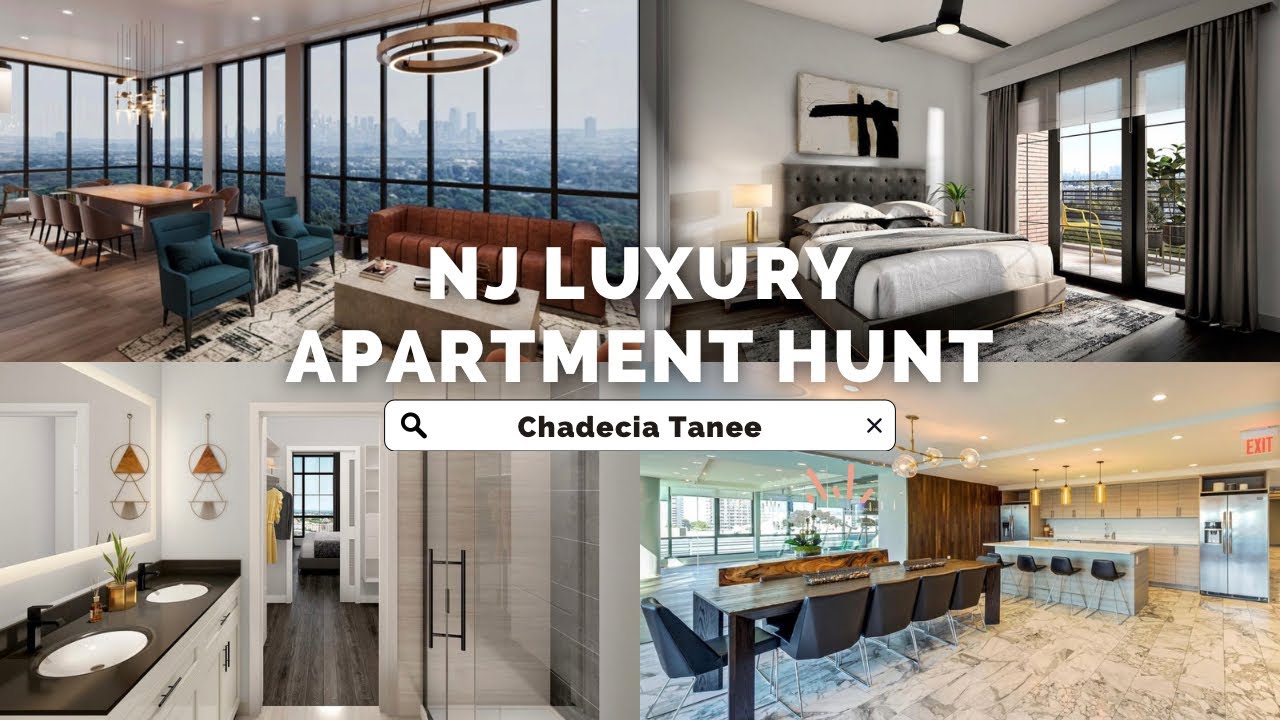**New York Luxury Apartment Hunt: A Showcase of Opulent Living Spaces**

Explore the epitome of urban luxury living with this stunning New York apartment advertisement, featuring four exquisite properties each offering unique and lavish amenities. 

In the upper left quadrant, discover a breathtaking penthouse boasting floor-to-ceiling glass walls that provide a panoramic view of the bustling city. The space is thoughtfully designed with premium dining tables and versatile seating areas ideal for both dining and meetings. 

Adjacent to this, find an expansive open-plan living room adorned with contemporary furnishings, including sleek chairs, a cozy throw rug, and a stylish coffee table. This area seamlessly blends indoor and outdoor living, thanks to the large glass doors leading to an inviting patio. 

The bedroom, flooded with natural light from the glass wall doors, offers direct access to the patio, ensuring a harmonious blend of comfort and luxury. It features elegant curtains that provide the option of complete privacy. 

The apartment includes a spacious, modern bathroom equipped with dual sinks and a luxurious shower, catering to every convenience with style. 

Completing the tour is a state-of-the-art kitchen area, highlighted by ultra-modern tables and chairs that speak to the elegance and sophistication of the entire space. 

This exceptional apartment promises an upscale living experience, undoubtedly commanding a significant investment reflective of its premium offerings.